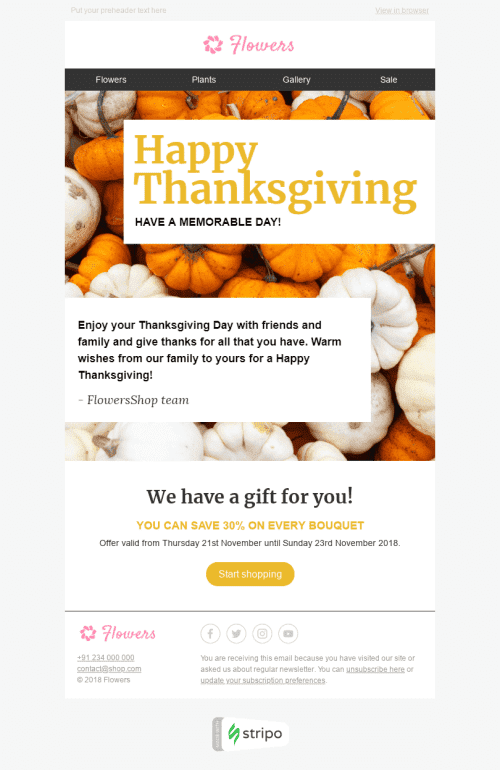This promotional email from a flower shop is themed for Thanksgiving and designed with a visually appealing and festive layout. The header prominently features the word "Flowers" alongside the shop's logo. Navigation links to various sections such as "Flowers," "Plants," "Gallery," and "Sale" are also included in the header for easy access.

The main message of the email centers around a cheerful "Happy Thanksgiving" greeting, complemented by the subtext, "Have a memorable day." Below this, there is a warm and heartfelt message encouraging customers to enjoy Thanksgiving with loved ones and to be grateful for all that they have. The email conveys warm wishes from the shop's team, stating, "Warm wishes from our family to yours for a Happy Thanksgiving. Flowers Shop Team."

A notable feature of the email is a special promotional offer, which states, "We have a gift for you. You can save 30% on every bouquet." The offer is valid from Thursday, November 21st until Sunday, November 23rd, 2018. To facilitate easy shopping, there is a prominent yellow button labeled "Start Shopping."

The footer of the email includes contact information, such as a phone number and email address, as well as social media icons for Facebook, Twitter, Instagram, and Google Plus. It also contains a legal notice indicating that the email was sent to recipients who have visited the site or requested newsletters, with links provided to unsubscribe or update subscription preferences. The email concludes with the Flowers logo and a copyright notice, "© 2018 Flowers."

While the email is effective in communicating Thanksgiving wishes and promoting a special offer, a suggestion is made that future communications should shift focus towards the upcoming Christmas season.